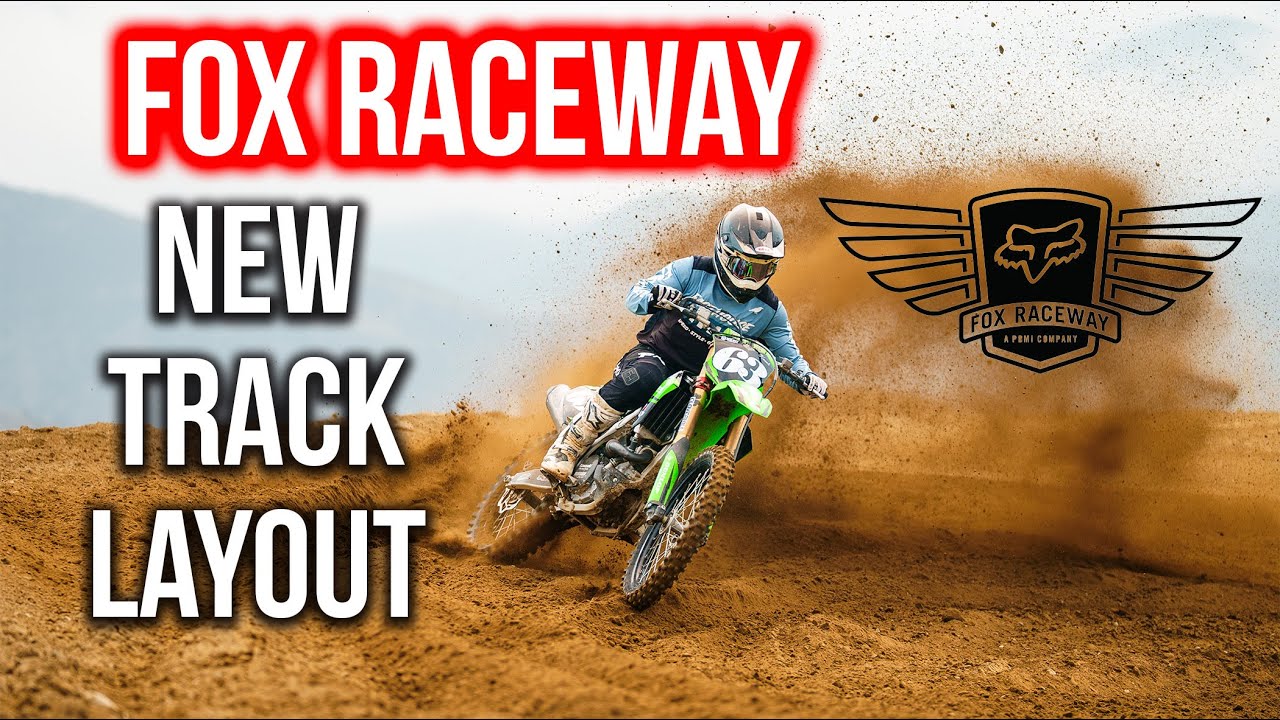The image looks like an advertisement for Fox Raceway, featuring a dynamic photo of a dirt bike rider navigating through rough, dirt terrain, and kicking up a cloud of dust behind them. The rider, wearing a light blue shirt and a black helmet, making their gender unclear, leans into a sharp turn on the green, mud-splattered bike numbered 63. At the top left corner, bold white text with a red glow states "Fox Raceway," while below it, the words "New Track Layout" are styled with a black shadow. Additionally, on the right side of the image, where the dirt is being kicked up, there's a detailed logo for Fox Raceway, displaying the name along with wings on either side, and identifying it as a P-B-M-I company.